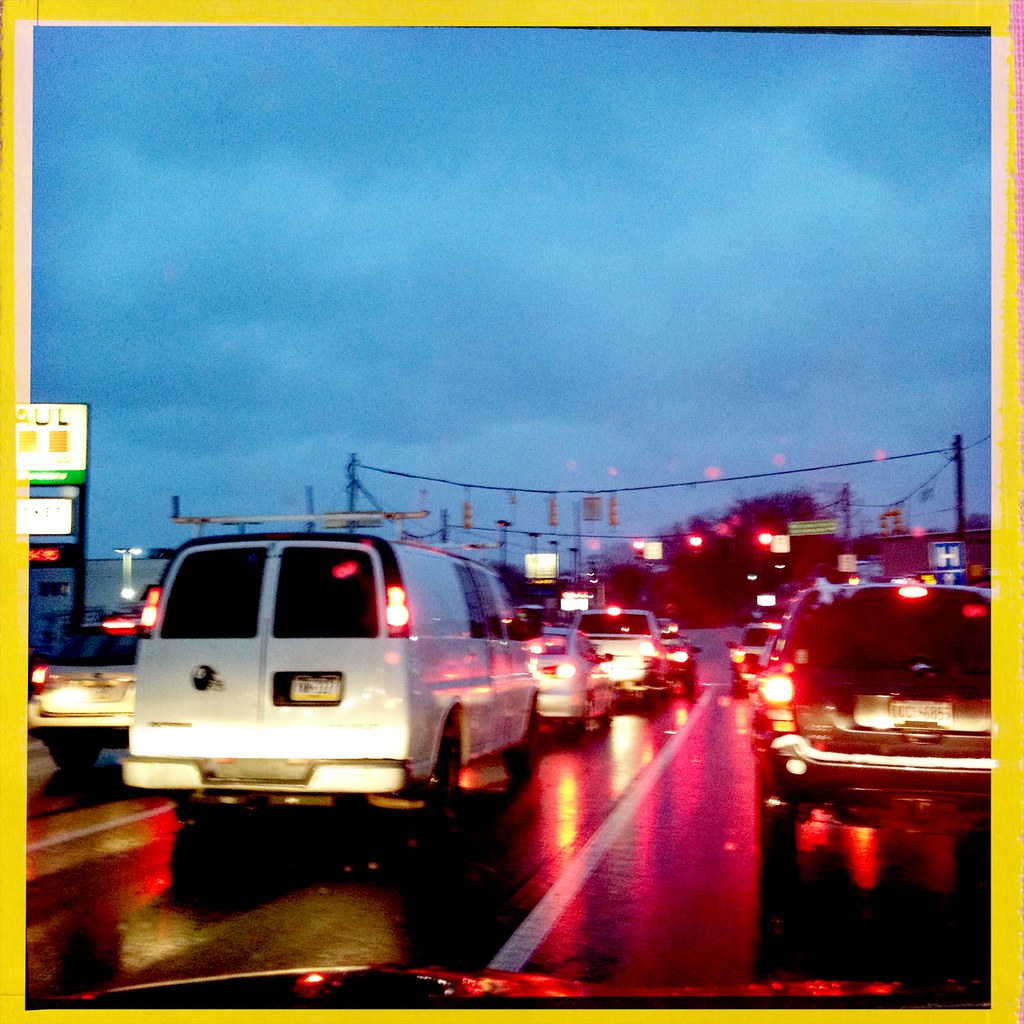Captured at dusk, this image vividly portrays a congested urban scene from the perspective of a driver. The sky is heavily overcast, casting a somber tone over the landscape. A multitude of vehicles can be seen waiting at a traffic light, their headlights and taillights reflecting off the wet asphalt in a dazzling array of colors. The road is glistening with moisture, enhancing the luminescence of the lights. 

In the foreground, four cars are lined up in the left lane, while several others are positioned directly ahead of the photographer's vehicle. A large pole stands tall, supporting an intricate array of traffic lights that stretch across the entire intersection. On the left side of the frame, a significant portion is occupied by a white van, obscuring a clear view of the traffic in the opposite direction. However, an array of lights on the left implies considerable activity.

Additionally, a blue hospital sign, marked with the characteristic white "H", is visible, signaling the presence of medical facilities nearby. Despite the heavy traffic, the scene is eerily calm, encapsulated by the moody twilight and the persistent drizzle, which together create a reflective, almost cinematic atmosphere.